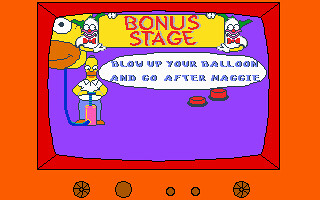This image is a detailed still from a Simpsons video game featuring a vibrant and whimsical design. The central focus is a TV-like screen with a bright orange outer border. The screen has a thin top border and thicker side borders with various knobs at the bottom: five brown buttons of different sizes, including two larger ones with textured designs and three smaller ones between them.

Inside the TV screen, there's a red inner border surrounding a purple background. At the top, a yellow banner with red lettering reads "BONUS STAGE," flanked by two images of Krusty the Clown with his green hair, white face, and red bowtie. Krusty appears to be holding up the sides of the banner.

In the middle left of the screen, Homer Simpson is depicted blowing up a balloon shaped like his own head using a blue-handled pump with a pink base and a blue hose. Homer, dressed in his typical white shirt, blue pants, and brown shoes, looks down at the pump while pushing its handle. Above him, a large white thought bubble states, "Blow up your balloon and go after Maggie."

To the right of the screen are two red buttons, adding to the game's interactive elements. This vivid and colorful still captures the playful and chaotic spirit of The Simpsons video game scene.